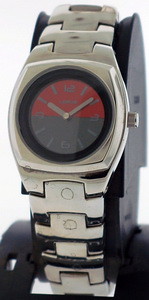The image showcases a sleek metal wristwatch elegantly displayed on a custom black plastic stand against a minimalist, featureless grey background. The sophisticated wristwatch, fastened securely around the stand, boasts an articulated metal strap with interlocking segments. The watch's dial is a distinctive curved square, containing a black face adorned with a striking concentric circle design. This circle is divided into two semicircles: the upper half in bold red and the lower half in a deep blue. The watch features grey hour and minute hands, meticulously pointing to a dial marked only by the numbers 3, 6, 9, and 12, while the remaining positions are denoted by minimalist lines. The stand is designed to complement the watch, ensuring that it stands upright and is showcased in its full glory.